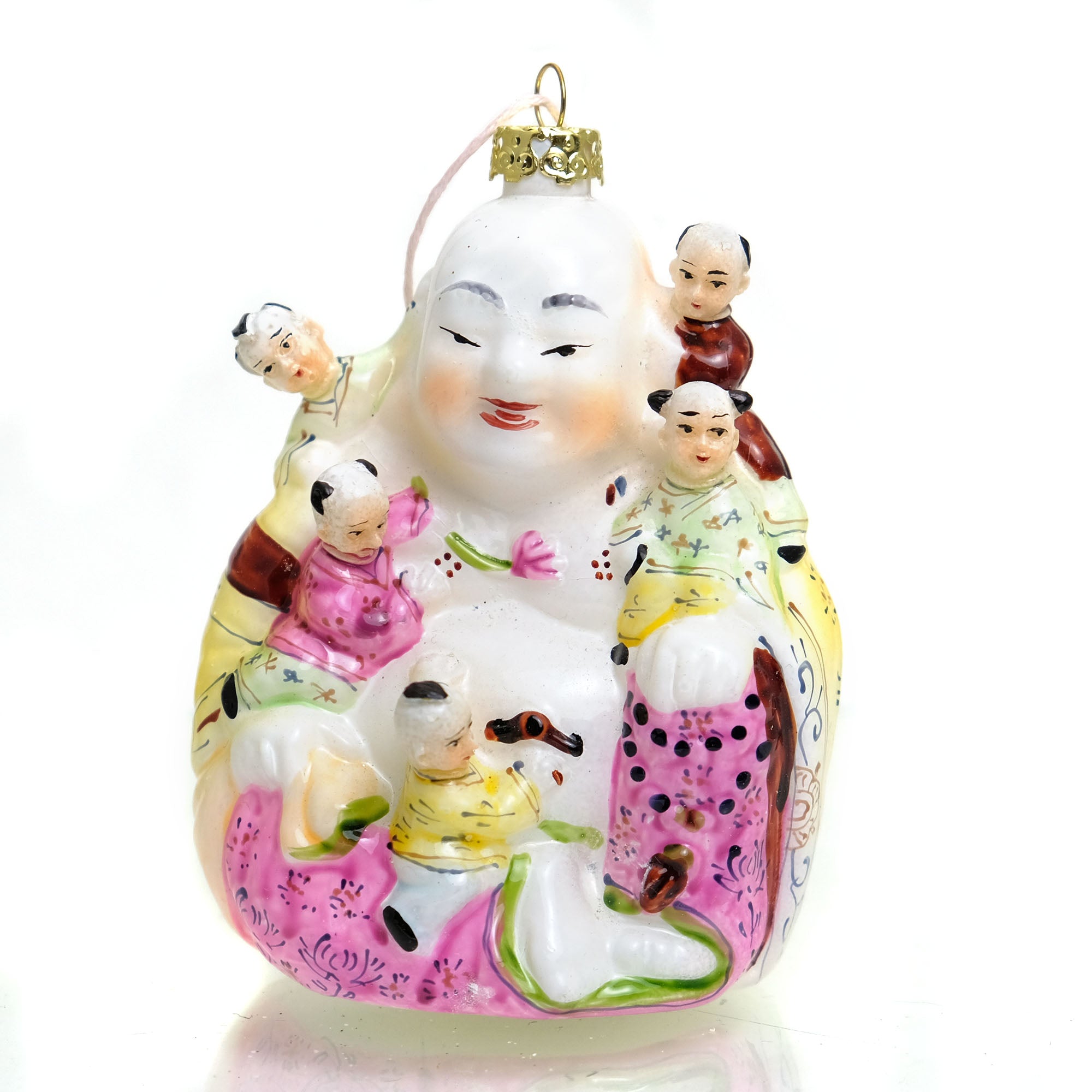The image portrays a large, intricately detailed Christmas ornament featuring a white porcelain figure of an Asian-looking Buddha with a big, round, white head and red lips. The Buddha, smiling serenely, is adorned with a yellow and pink robe with floral accents, revealing a slightly exposed belly. Surrounding the Buddha and intricately attached to its form are five small children, each with distinctive bald spots in the middle of their heads and small tufts of hair on the sides. Two children cling to the Buddha's ears, two are positioned on its chest, and one encircles its belly. The ornament has a classic golden cap and hoop at the top, complete with a rope likely meant for hanging on a tree. The backdrop of the image is stark white, emphasizing the finely painted detail and colorful accents on the ornament.